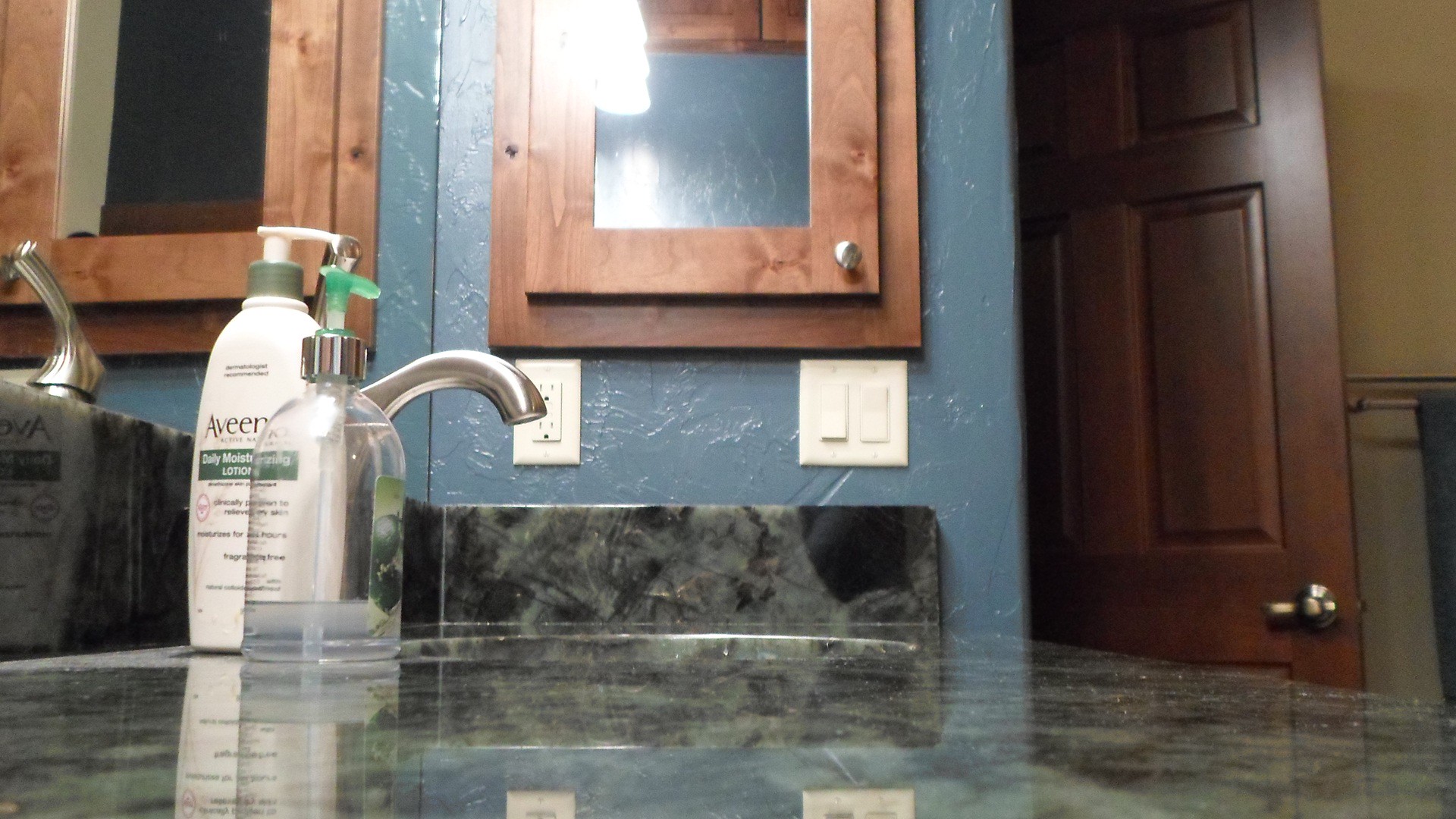In this detailed photograph of a bathroom, the camera is positioned on the black and gray marbled sink surface, capturing an encompassing view. The image showcases a lavishly designed space, highlighted by a solid cherry oak bathroom door with a decorative, high-end handle that gleams under the ambient light. The walls are painted a warm yellow, providing a cozy contrast to the sleek, silver towel rod that supports a neatly hung blue towel. 

On the sink countertop, the highly reflective surface mirrors the adjacent white light switches, adding depth to the composition. Prominently placed on the sink is a green and white Aveeno moisturizing lotion bottle, clearly labeled. Beside it, a nearly depleted, clear glass soap dispenser with a green spout adds a touch of functionality to the scene. 

The large mirror above the sink provides an expansive reflection of the bathroom, further emphasizing the room's sophisticated decor. On the side of the sink, a wooden medicine cabinet with a circular silver pull and an additional mirrored front offers practical storage while enhancing the room's elegant design. Overall, the image captures a well-appointed bathroom, exuding both luxury and practicality.